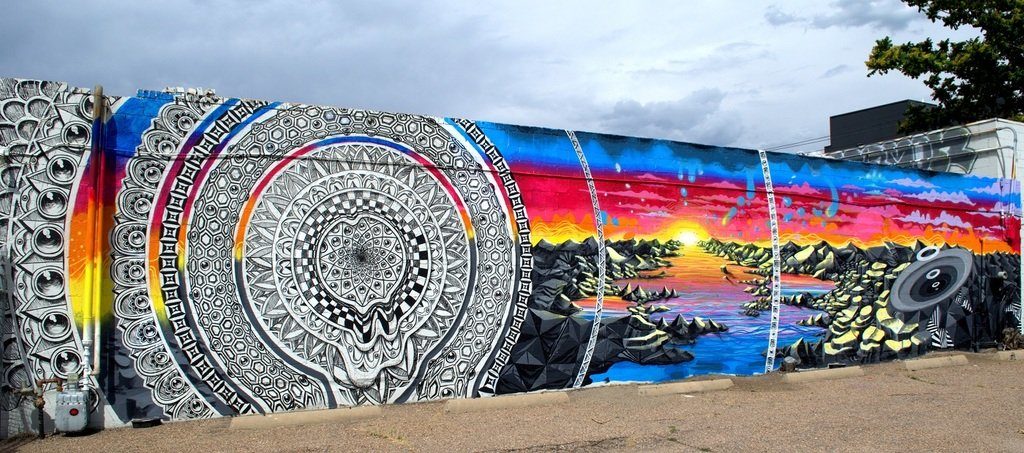This image captures a sprawling mural painted on a concrete wall, potentially the back of a single-story building adjacent to a gravel parking lot. The mural extends from ground level to the top of the wall and features a complex, abstract design that transitions from left to right. 

On the left side, the mural displays intricate black-and-white geometric patterns, including concentric rings with various pointy and circular elements, reminiscent of a Mayan calendar. These rings, adorned with little circles and angular designs, appear to float apart as they radiate outwards. Moving to the right, a vertical strip composed of blue, pink, orange, yellow, and blackish-gray hues divides the mural, adding a colorful contrast. 

Central to the mural is a large metal-colored circle with numerous smaller circles, evoking the appearance of mechanical components or eyeballs. This segment is surrounded by a vibrant backdrop featuring the aforementioned colors and metallic elements. 

Further right, the mural transitions into a serene landscape scene. A river, flanked by rocks, meanders into the background under a striking sunset. The sky above the river is painted in hues of pink, red, and blue, with a reflection of the sun creating a path of light along the water. The entire scene is underpinned by a sense of tranquility and abstract beauty, culminating in a vivid narrative that blends mechanical precision with natural splendor.